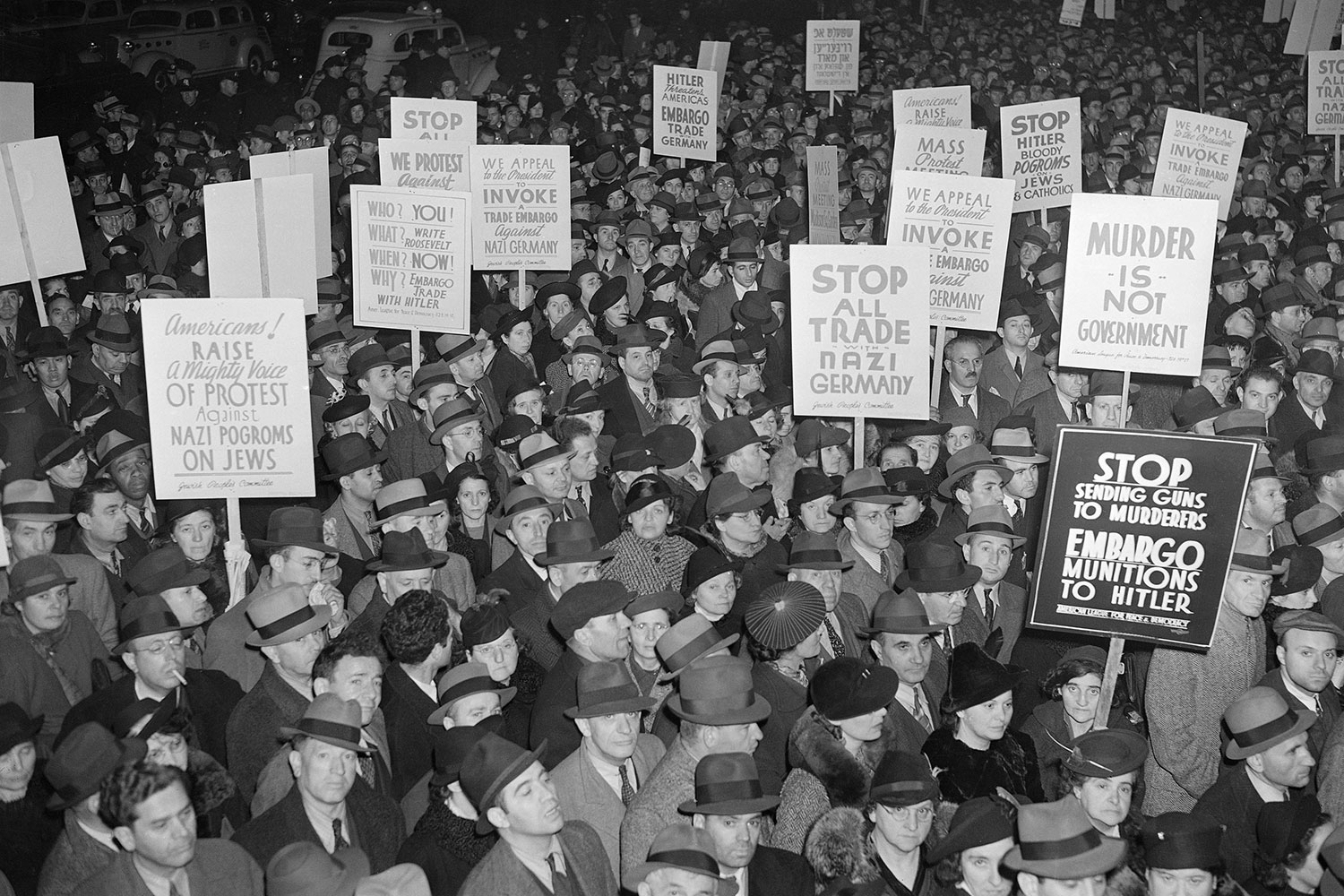The image is an old black-and-white photograph, likely taken in the 1930s during the World War II era, depicting a nighttime protest. The scene shows a massive throng of people, standing shoulder-to-shoulder, filling the frame. Most of the protesters are men dressed in suits, long coats, and brimmed hats, while the women, who are fewer in number, are elegantly dressed in fur coats and hats. The crowd is predominantly male, but the presence of women is notable. 

Many of the protesters are holding signs with stark messages. The slogans on these signs read, "Stop all trade with Nazi Germany," "Murder is not government," "Stop sending guns to murderers," "Embargo munitions to Hitler," and "Americans raise a mighty voice of protest against Nazi pogroms on Jews." Some signs are white with gray writing, while others are black with white writing, making the messages stand out in the dim lighting. 

In the top left corner of the photograph, a few old Packard-looking cars are visible, adding to the historical context of the scene. The crowd appears tightly packed, with an estimated hundreds of people engaged in the protest, vividly capturing a moment of widespread dissent against Nazi Germany's policies and actions.